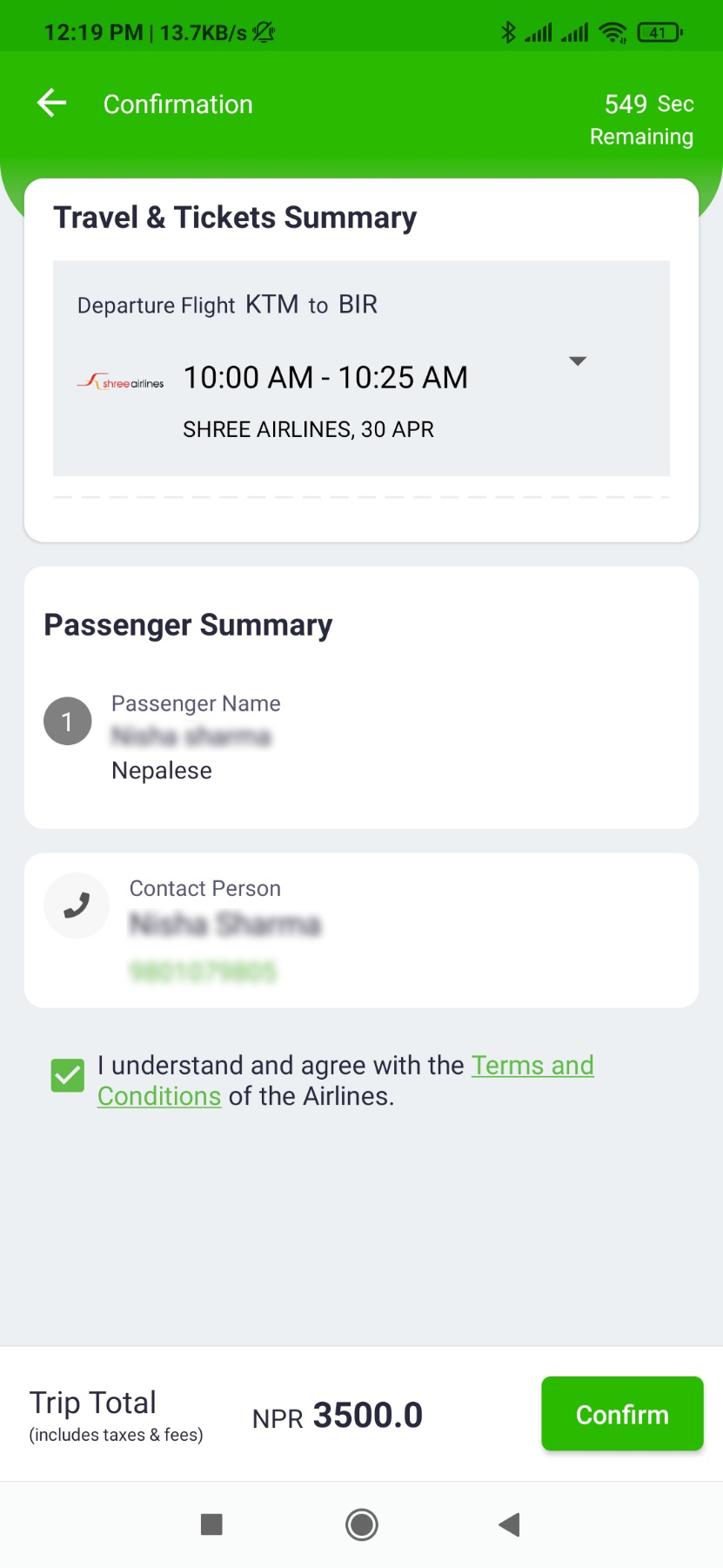In the screenshot taken from a mobile device's website or app, the image begins with the information bar at the top of the screen. On the left-hand side of this bar, the time is displayed as 12:19 p.m., followed by the data speed of 13.7 KB/s. Adjacent to this is a bell icon with a strikethrough, indicative of either a muted notification or sound setting. Further along the top bar, the Bluetooth symbol is visible, followed by two Wi-Fi signal strength bars, a cellular signal strength icon, and a battery indicator showing 41%.

Below the information bar is the title bar labeled "Confirmation," featuring a back arrow on the left and "549 seconds remaining" on the right-hand side. Directly beneath the title bar, the "Travel and Ticket Summary" section provides details of a departure flight from KTM to BIR, scheduled from 10:00 a.m. to 10:25 a.m., operated by Sri Airlines on the 30th of April, with a drop-down arrow beside it for further details.

Subsequently, the "Passenger Summary" section states there is one passenger, whose name is blurred out, and identifies their nationality as Nepalese. Below this, a phone icon accompanies the label "Contact Person," with the blurred name and phone number, barely legible but appearing to read "Nisha Sharma."

Towards the end of the image, a checkbox affirms the agreement with the airline's terms and conditions and is marked as checked. Finally, at the bottom of the screen, the trip's total cost, inclusive of taxes and fees, is noted as NPR 3,500, positioned next to a prominent "Confirm" button.